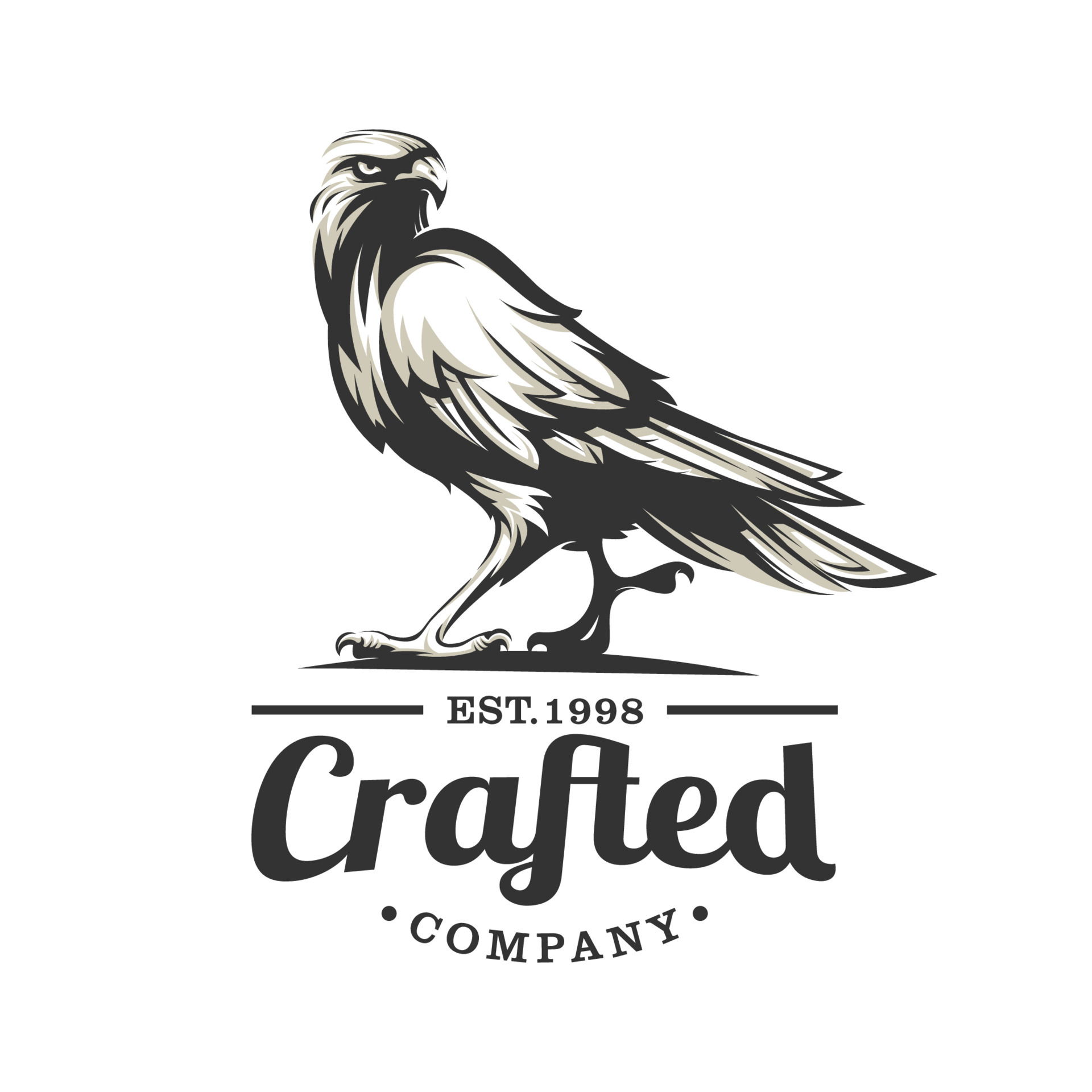The image depicts a monochromatic company logo for Crafted Company. Dominating the center is a black and white illustration of a powerful bird, reminiscent of an eagle or falcon. The bird's fierce eyes and sharply defined lines exude an intimidating presence as it gazes over its shoulder, standing firmly atop a shadowed base. Below this striking avian figure, the logo features "EST. 1998" flanked by thin lines, followed by the word "Crafted" in a semi-cursive font. The word "Company" appears beneath in bold, standard print, punctuated by dots on either side. The overall design maintains a stark black and white color scheme set against a pure white background, underscoring the brand's refined and classic aesthetic established since 1998.